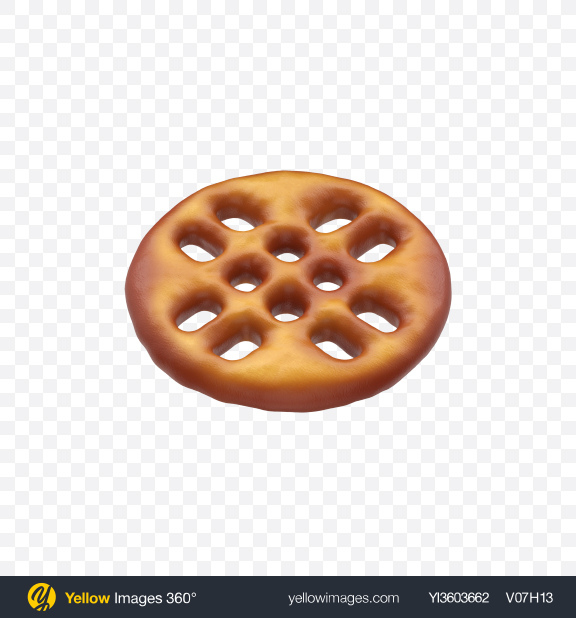The image depicts a detailed computer rendering of a biscuit, resembling a Ritz cracker, centered on an alpha grid background characterized by an alternating pattern of white and light gray squares to indicate transparency. The biscuit itself is a circular, golden-brown treat with a distinctive design. It features four round holes arranged in a diamond shape at the center, surrounded by four extended oval shapes radiating outward, forming an X pattern. Below the biscuit, a black horizontal bar spans the width of the image. The left side of this bar contains a small yellow icon followed by the text "Yellow Images 360 degrees" in yellow and white. Further to the right, the bar displays the URL "yellowimages.com" and a serial code "YI-360-3662-V-07-H-13" in white text, spaced evenly across the bar.